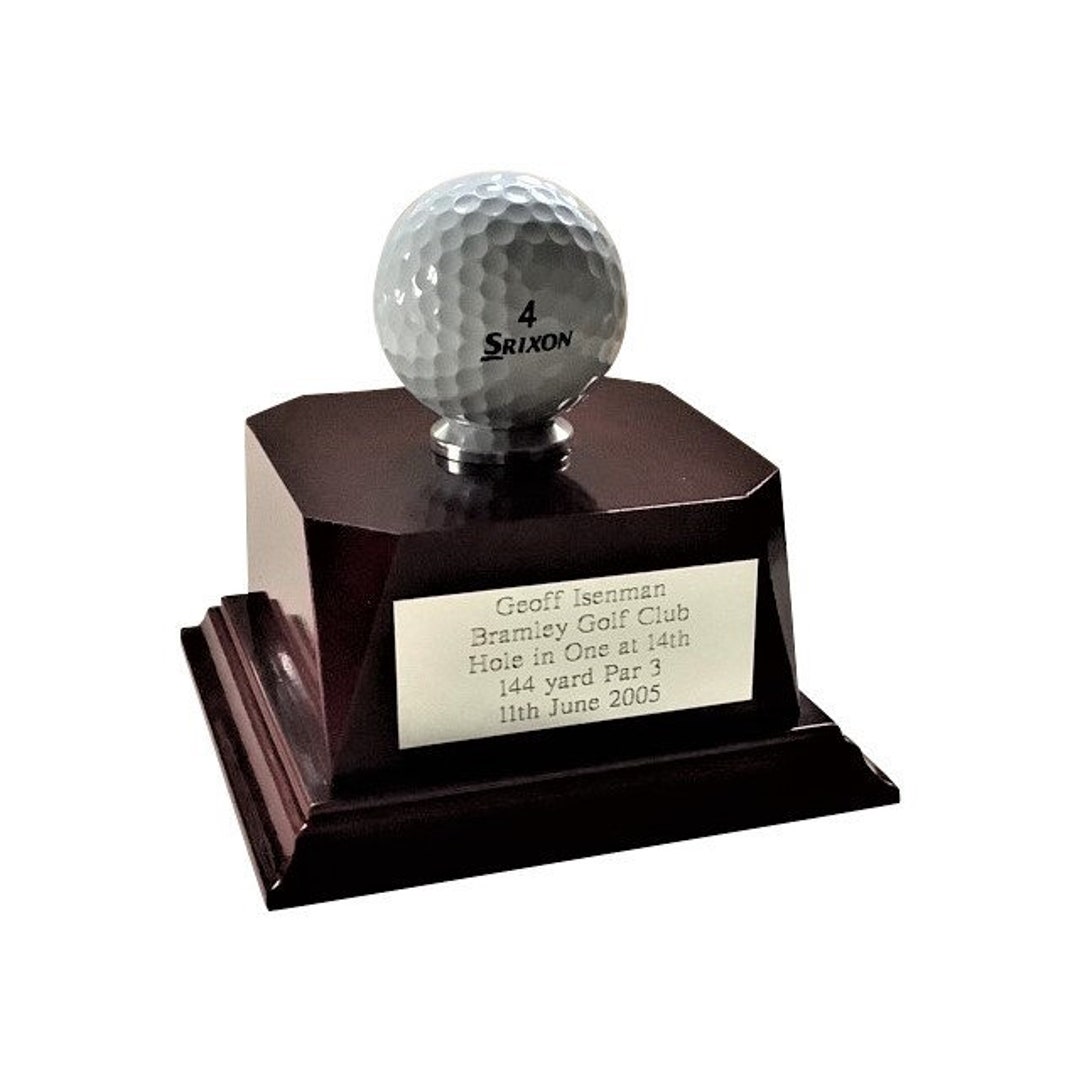The image is a color photograph with a white background, featuring a small, shiny golf trophy. The trophy is crafted from dark wood with clipped corners and has a square shape. Mounted on a silver circle at the top of the wooden base is a white golf ball with black text, displaying the number 4 and the logo "Srixon." Beneath the golf ball, a gold rectangular plaque is attached to the front of the wood base, engraved with the following details: "Jeff Eisenman, Bramley Golf Club, hole in one at 14th, 144 yard, par 3, 11th June 2005." The trophy is presented at a slight angle, with the left side lower than the right, creating a dynamic visual effect.